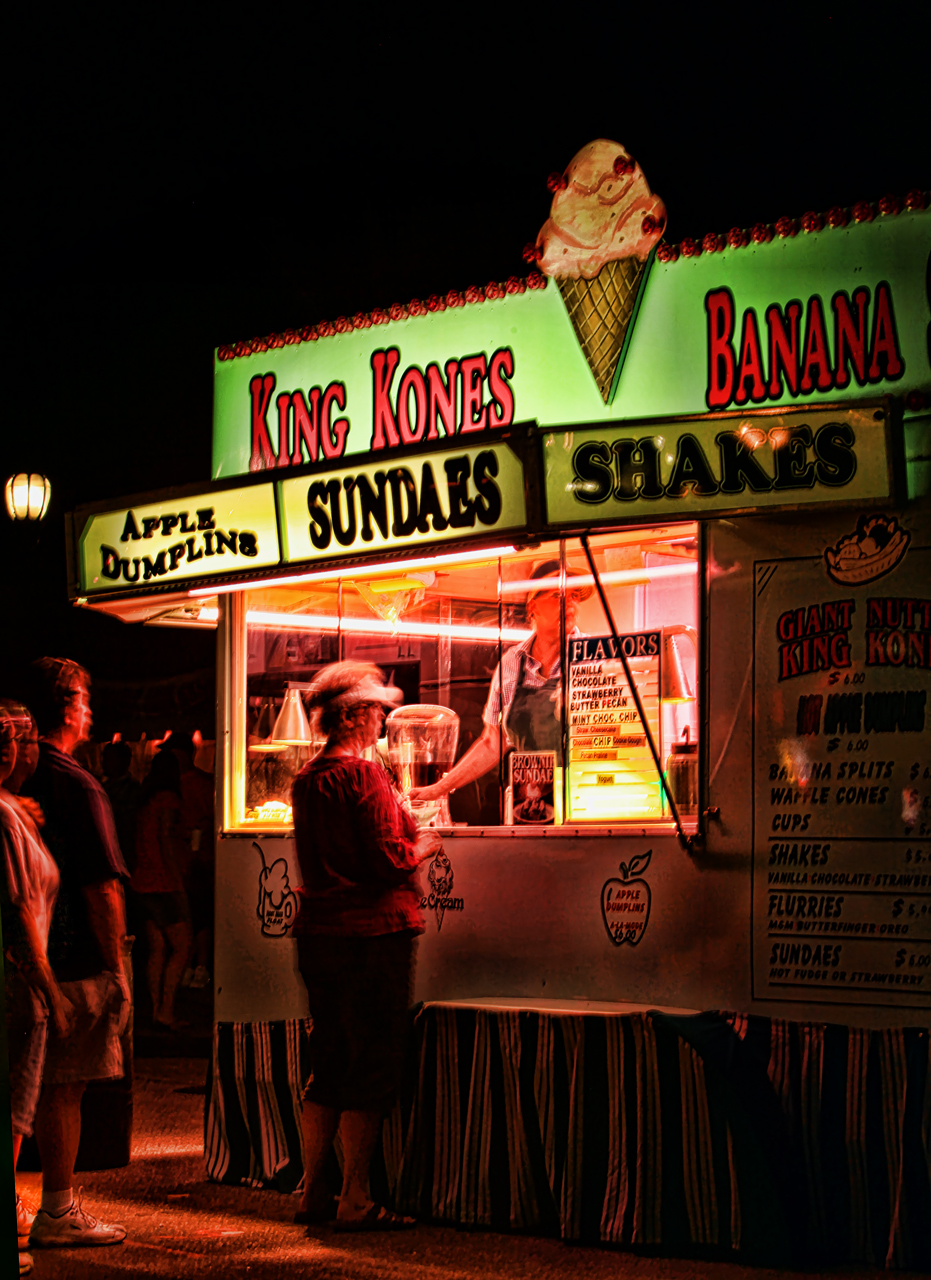The photograph captures a bustling nighttime scene at a vividly lit food trailer, specifically an ice cream stand known as "King Cones." The trailer is adorned with a distinctive black and yellow striped skirt at the bottom, concealing the wheels. Above, the trailer is a white metallic box with windows on its side and back. Prominent, backlit signage crowns the trailer with a striking green logo that reads "King Cones" in bold red text with black borders. This logo is flanked by the word "Banana" and features a large, stylized brown waffle cone topped with a pink scoop of ice cream. 

Below the main sign, another illuminated overhang displays a series of yellow squares that advertise "Apple Dumplings," "Sundaes," and "Shakes." The serving window is situated on the left side of the trailer, with an extensive menu visible on the right. The scene is animated by the presence of several patrons: a person stands at the window placing an order, and a small queue forms behind them, with additional people faintly discernible in the darker background, hinting at the lively atmosphere. The lower half of the photo is tinted red, adding to the vibrant, nighttime ambiance of this popular ice cream destination.